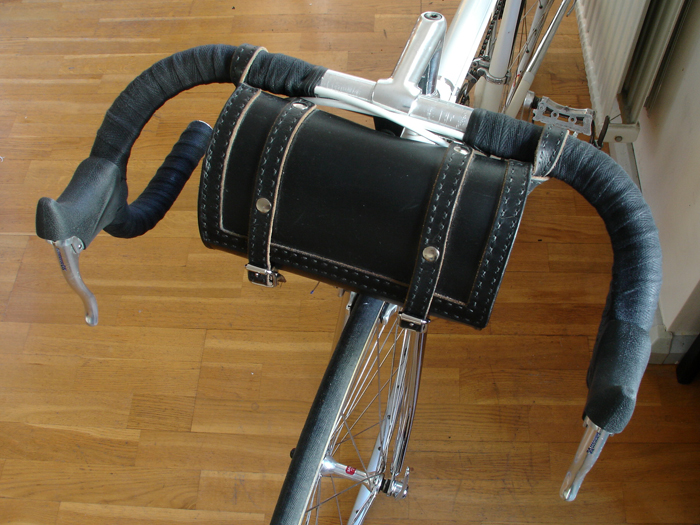The image captures an indoor scene featuring the front portion of a silver and black bicycle. The bicycle's handles are wrapped with black tape and equipped with brakes, while a small black leather bag with gray or tan stitching is attached to the handles. The bicycle is positioned on a brown wooden floor, with a tan wall in the background, complete with baseboard molding at the bottom. Towards the upper part of the image, there's a partially visible window treatment, possibly curtains or shades, in a tan color with gray and black in the center. The photograph highlights the front wheel and part of the bicycle's gears, emphasizing the detailed indoor setting.